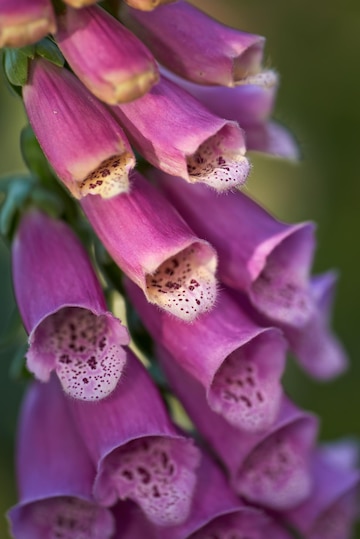This close-up photograph captures an abundance of small, purple, tube-like flowers resembling thimbles or trumpets. Each flower measures approximately an inch in diameter and three inches in length. Their interiors are mostly white with distinct dark purple splotches, giving them a speckled appearance. The flowers exhibit a bell-like shape, and their light purple petals are edged with a delicate, hairy texture. The green leaves at the base of the tubes are thick and dark, providing a contrasting backdrop that is pleasingly blurred. This ensemble creates a layered effect, with flowers and leaves overlapping each other, emphasizing the abundant and intricate nature of the plant.